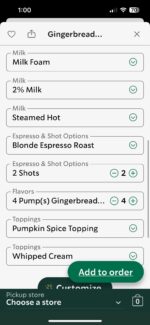This is a slightly blurry screenshot of a restaurant ordering screen. At the top of the image, there's a black banner displaying the time (one o'clock), a Wi-Fi symbol, and a battery indicator. Below the banner, a prominent white pop-up with black text is visible. At the top of this pop-up, there is a black heart icon and a black box with an arrow, alongside the text "Gingerbread..." and a gray 'X' for closing the window.

Further down, a list of customizable options is presented in white boxes with black text. Each option features green icons next to them. The options include:

- **Milk Options**:
  - Milk foam
  - 2% Milk
  - Steamed Hot Milk

- **Espresso and Shot Options**:
  - Blonde Espresso Roast
  - Two Shots (with a plus and minus sign for adjustment)

- **Flavors**:
  - Four pumps of Gingerbread (indicated by a black number 4)

- **Toppings**:
  - Pumpkin Spice Topping
  - Whipped Cream

Next, there's a "Customize" button inside a forest-green box with white text. Below this are two additional green boxes; one says "Add to Order," and the other, "Pick Up Store," accompanied by the text "Choose a Store" and a drop-down arrow for selection. There is also a shopping bag icon showing a count of zero items.

Finally, a thin white line borders the bottom of the screenshot. Despite the image's blurry quality, the details of the order screen's interface are discernible.